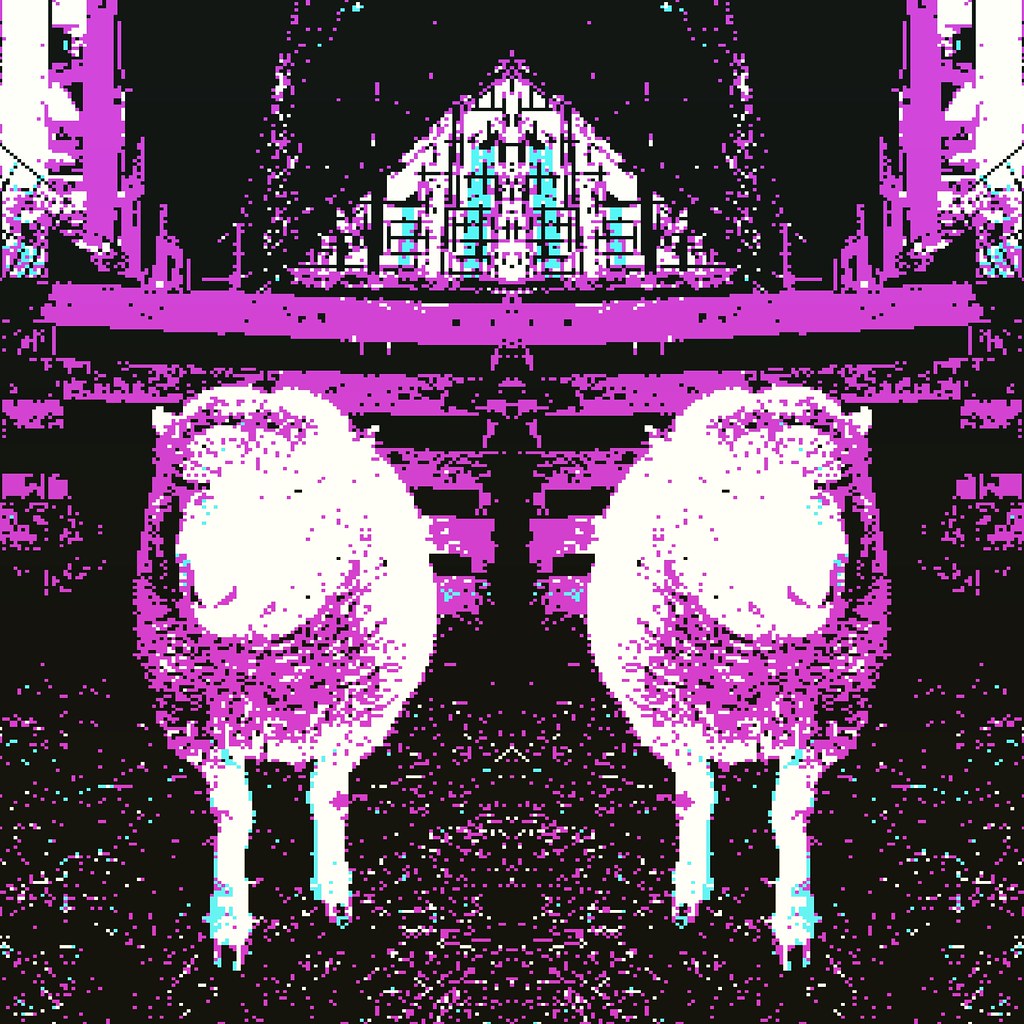The image presents a unique artistic rendering of two sheep, appearing side-by-side and seemingly mirrored to look like twins. The scene is highly pixelated, lending a retro video game aesthetic reminiscent of early Nintendo graphics. The color palette is limited to vibrant neon pinks, purples, whites, baby blues, and blacks, creating an overexposed, almost negative-like effect. Each sheep is depicted through dense clusters of pink and white dots, with shades of purple and black adding depth to their forms. They stand in front of a somewhat indistinct background that appears to comprise wooden planks, possibly representing a fence or gate. Above them, a triangular structure—potentially part of a stained glass window or an A-frame—adds to the surreal backdrop. The ground below them is black, speckled with colored dots, contributing to the overall pixelated and glitter-like texture of the image.